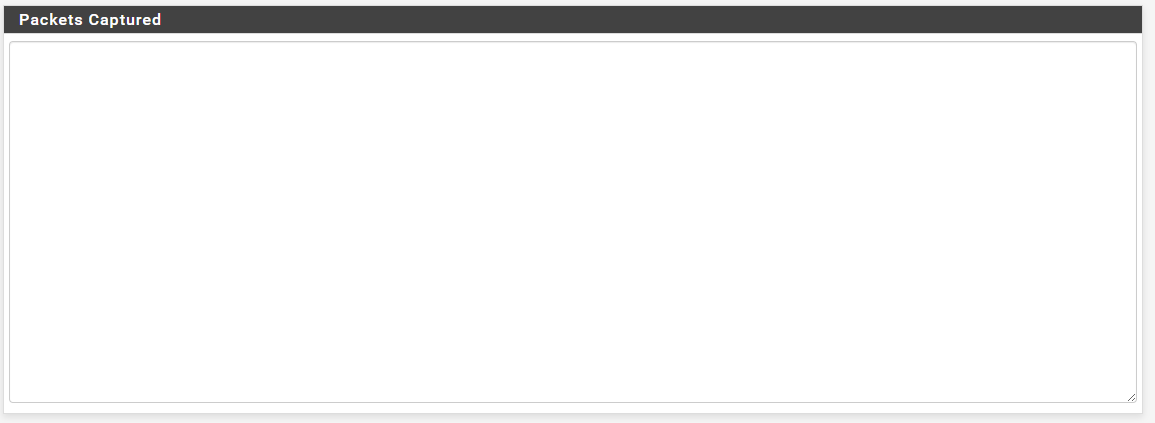The image depicts a simple interface with a high visual quality. At the top of the image, there's a prominent, large rectangular box. This box features a long black strip at the very top, displaying the text "Packets Captured" in a bold white font. Notably, the 'P' in 'Packets' and the 'C' in 'Captured' are capitalized, ensuring high readability. Below this black strip, the rectangle primarily consists of a large, empty white space, framed by a thin gray outline. At the very bottom corner of this white box, there's a faint black mark. On the right side of the image, there appears to be a partial view of a scroll bar, indicating that this might be part of an interactive site or form for entering information. The image is crisp with no pixelation or blurring, although there are slight shadows visible. The overall quality remains high, despite the minimalistic content and lack of additional text or images.